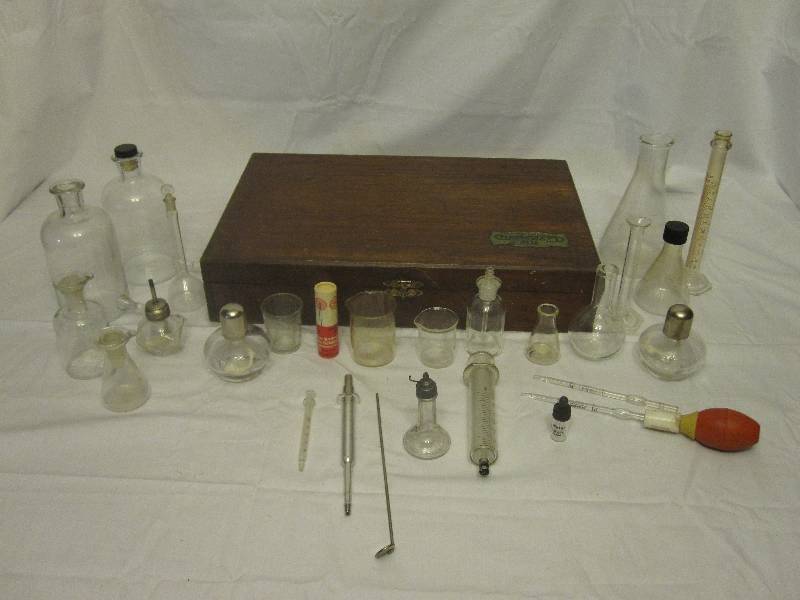The image depicts an indoor setting with photographic clarity, featuring an array of scientific glassware arranged on a wrinkled white tablecloth. Centered in the background is a brown briefcase with a gold buckle and emblem; the emblem's black text is not discernible. From left to right, the glassware lineup begins with two tall glass bottles, around 12 inches high—one with a black stopper and the other open. These are followed by two smaller glass bottles, about 6 inches tall each, one of which features a spout-like tip. Continuing to the right, there is a small globe-shaped glass, a regular drinking glass, and a red and white cylinder-shaped shaker with distinctive writing. Next are more glasses, including one with a stopper and another small flask, followed by a thin-necked flask and a tall cylindrical flask. The collection also includes a bulb-shaped glass with a silver top and two triangular flasks—one with a black top, the other standing about 14 inches tall. A graduated cylinder marks the end of the lineup.

In the foreground, various metal and glass tools associated with medical or laboratory use are scattered. Among them are what appears to be a dental mirror, a metal syringe, a suction pump, and a bulb attached to a long cylinder. All items are meticulously placed, emphasizing the science-themed ensemble against the simple yet textured backdrop.